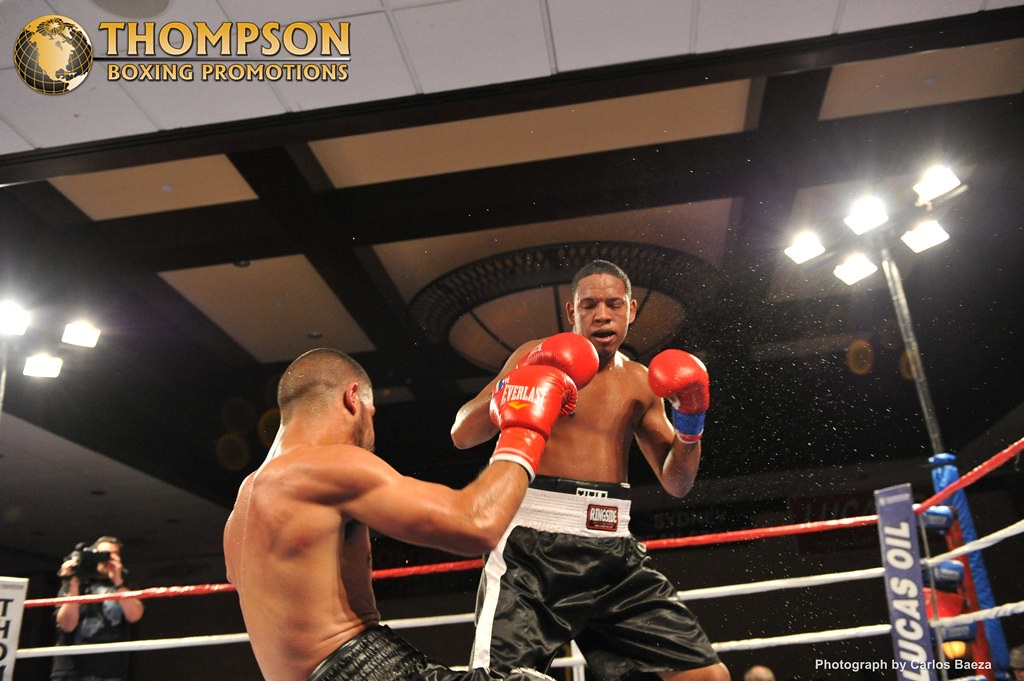The image is a detailed color photograph, captured in a landscape orientation, depicting an intense moment in a boxing match between two African-American men. Both boxers are shirtless, sporting black satin trunks and distinctive boxing gloves—one pair entirely red and the other red and blue. The scene unfolds in a well-lit boxing ring featuring three ropes: two white and one red.

The central focus is on the boxer who remains standing. He has very short hair and is clean-shaven, wearing orange gloves with a white band at the waist of his black trunks. He gazes down at his opponent, who appears to be falling, his back partially turned toward the camera, revealing a shaved head. This boxer wears orange gloves with the white Everlast logo.

Surrounding the ring, the atmosphere is electric, with scattered spectators visible in the dim background. Above the action, the ceiling is wood-toned and white, adorned with floodlights illuminating the scene. A logo in the top left corner reads "Thompson Boxing Promotions" in gold lettering next to a globe image. Additionally, the lower left corner captures a cameraman, documenting this intense moment. The ring's corner support also features "Lucas Oil" in bold white letters. The vividness and realism of the photograph capture the drama and energy of the boxing match vividly.